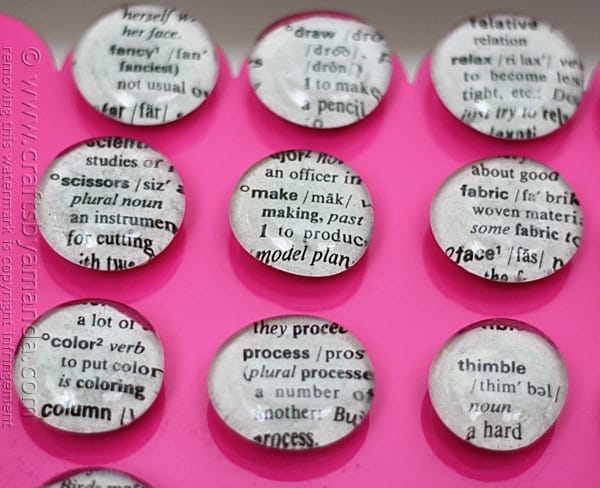The image features a pink background with a scalloped edge at the top, blending into a gray area above. In the lower left corner, there's a watermark that reads www.craftsbyamanda.com, cautioning against the removal of this watermark due to copyright issues. The centerpiece of the image displays nine round, translucent button-like objects that resemble clear pebbles or badges, arranged in a 3x3 grid. Each of these buttons contains a black font word on a white background, coupled with an explanatory text or definition, which appears to be cut out from a dictionary. The words are related to sewing and crafting, including "scissors," "fabric," "thimble," "process," "making," "draw," "relative," "relax," and "color." The translucent nature of the buttons gives them a water drop-like appearance, effectively showcasing the defined words beneath them.